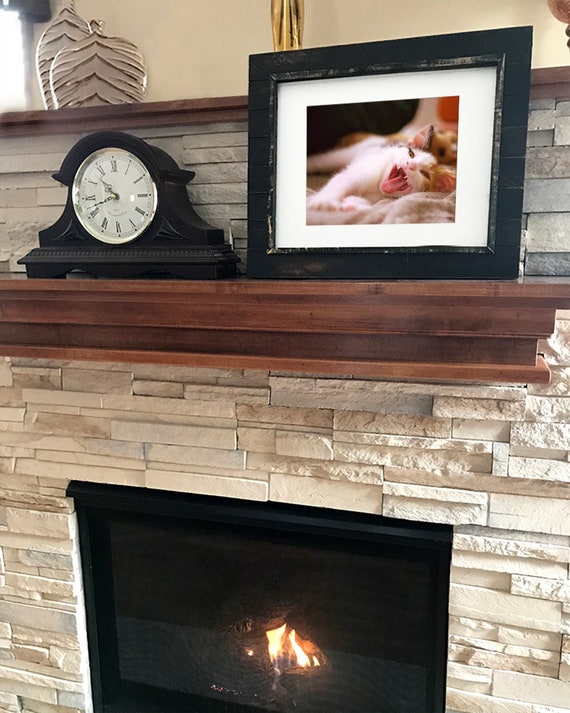This detailed color photograph, oriented in portrait format, captures an intricately designed fireplace setting. The fireplace itself features a cream-colored stack stone facade with a see-through black door cover. Inside, a lit fire casts a warm glow. Above the fireplace is a dark brown wooden mantel. 

On the mantel, positioned slightly to the left, is an elegant mantel clock with a black wooden frame and a white circular dial encircled by a chrome bezel, displaying Roman numerals. To the right of the clock is a framed photograph of a cat. The black-framed picture depicts a white cat lying down, stretching its paws forward, and yawning wide, with multicolored ears. The frame also includes a stone-colored tile detail and a white mat around the image.

The mantel itself supports additional decorative items, including white and beige-gold vases, adding a touch of sophistication to the scene. The entire setup is set against a white brick wall, contributing to the composition's visual appeal. The photograph, taken from a slightly off-centered angle on the right, emphasizes the carefully curated decor, presenting an inviting and cozy domestic atmosphere.